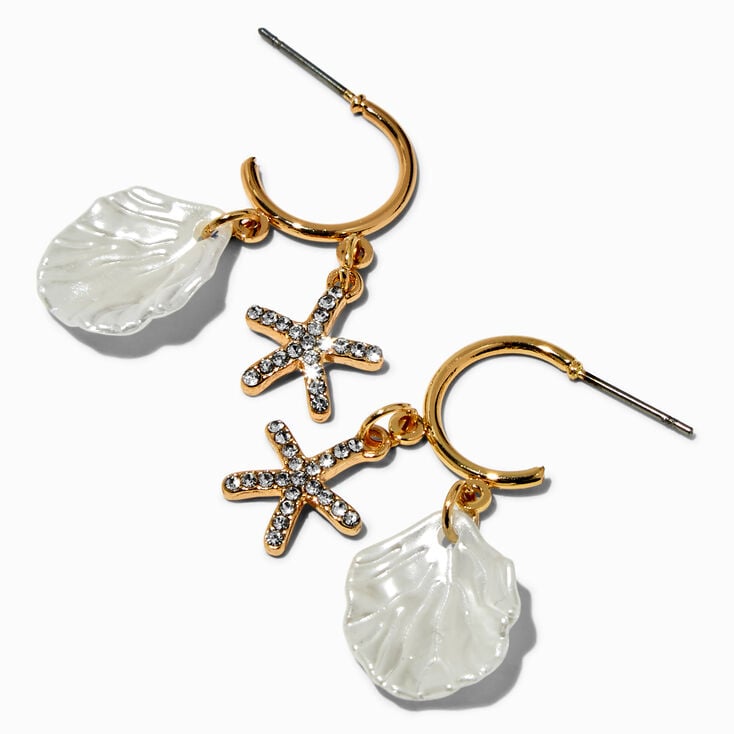This square-shaped image, approximately five to six inches in height and width, showcases a pair of elegant earrings displayed on a white background. Each earring, identical to the other, features a delicate design composed of a silver post for pierced ears leading to a gold C-shaped half loop. Dangling from each gold loop is a smooth, reflective white shell-shaped charm, possibly made from pearl or abalone, which captures and reflects light beautifully. Complementing the shell, each earring also displays a gold starfish charm adorned with small round diamonds along its arms, adding a touch of sparkle. The arrangement of the earrings in the image places one in the upper left and the other diagonally positioned to the lower right, enhancing their symmetrical elegance.